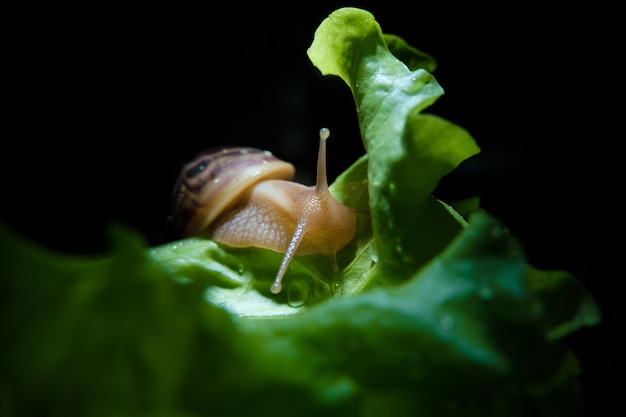This photograph, taken with a completely black background suggesting an indoor setting like a terrarium, features a snail climbing over a large, dewy leaf. The snail, with a slightly pinkish-tan, gelatinous body, is positioned to the left of the image, facing right. Its shell displays a blend of tans and blacks. The snail's two antennae are distinctly positioned, one extending upwards and the other bent downward. The leaf, which appears to be a piece of green lettuce adorned with water droplets, stretches upward in the center of the image, seemingly being nibbled on by the snail as it ascends. The detailed texture of the snail's body also reveals faint white marks, adding to the intricate details captured in this close-up, still-life photograph.